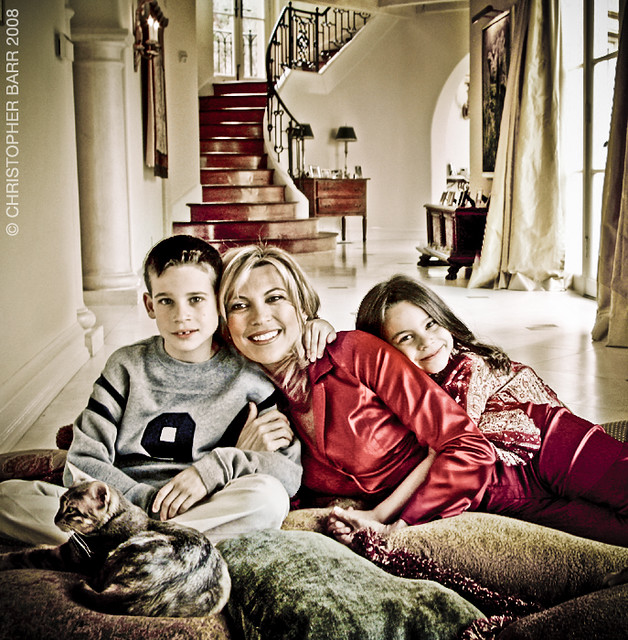This detailed family portrait of Vanna White, taken by Christopher Barr in 2008, captures an intimate and elegant moment with her two children and their tortoiseshell cat in the main entryway of their home. Vanna, who is positioned at the center of the photo, lies on brown and green floor pillows, wearing a red shiny blouse and smiling warmly. Her blonde hair cascades as she leans towards her son on the left, who is dressed in a gray sweater with a number on it, khaki pants, and has short dark hair. To Vanna’s right, her daughter, in a purple-pink outfit, rests her head on Vanna’s shoulder, gently hugging her back, with long dark hair flowing. The family cat poses in front of Vanna's son, looking to the left.

The background reveals an expansive, upscale room featuring a large curving stairway with a wrought iron railing, exuding an air of elegance. The stairway is bordered by a mirror or clock mounted on the wall. Other elements like tables, a chest, photos, lamps, large draped windows, and an open walk-through window contribute to the room's sophisticated ambiance. The tile floor further enhances the room's opulent style. At the upper left corner of the photo, the photographer's signature, "Christopher Barr, 2008," is subtly included, adding a personal touch to this beautifully composed image.